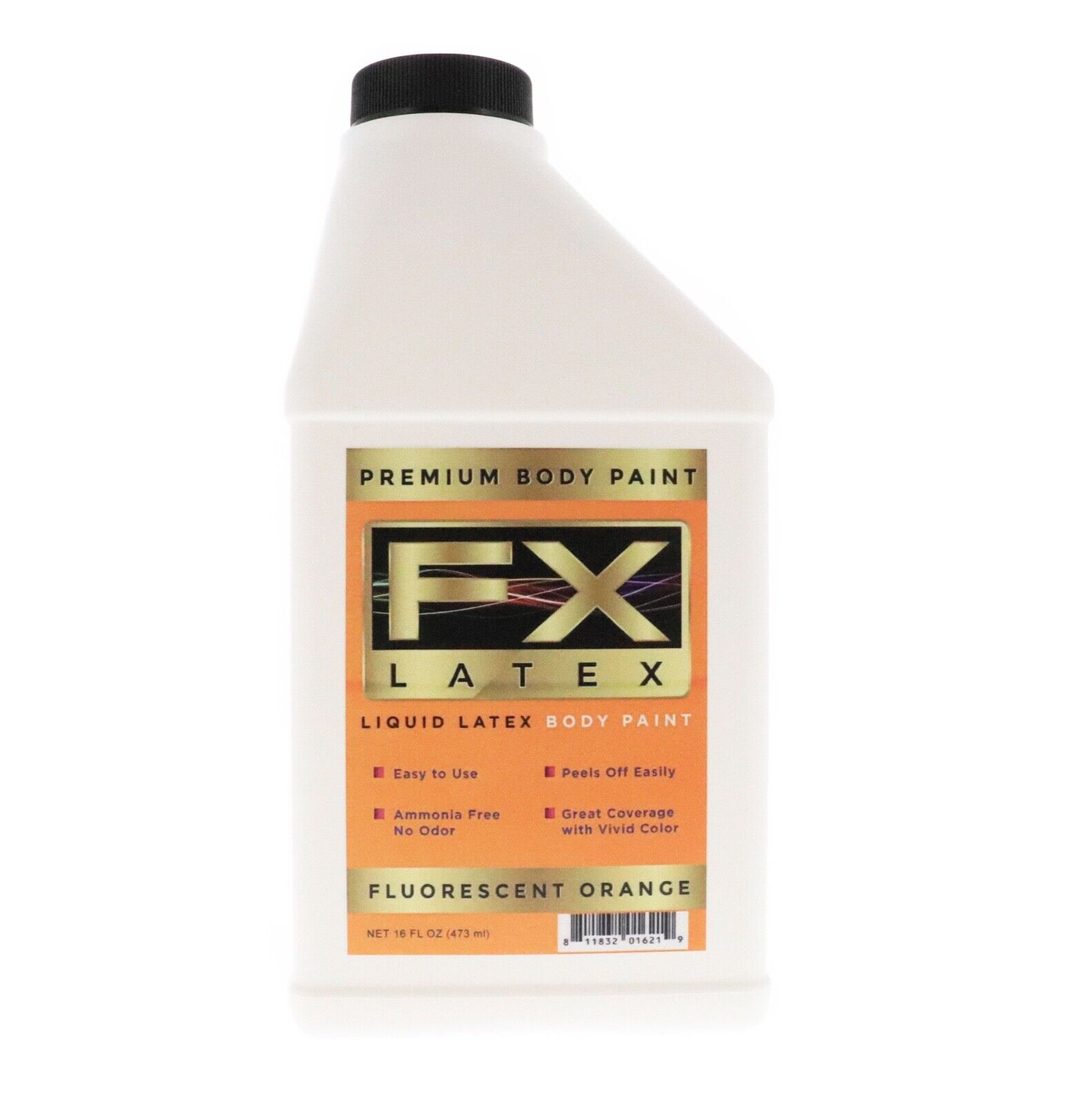The image features a close-up of a white container with a black screw top, set against a white background. The container sports an orange label with detailed gold and black text. At the top of the label, there is a gold rectangle enclosing a smaller black rectangle that prominently displays "FX" in large gold letters. Directly below, the text reads "premium body paint" and "latex" in black letters and beneath that, "liquid latex" in black followed by "body paint" in white. The label further lists four key product features in bullet points: "easy to use," "peels off easily," "ammonia-free, no odor," and "great coverage with vivid color." At the bottom of the label, against a gold strip, is the text "fluorescent orange" in black, along with the net weight of "16 fluid ounces (473 milliliters)" and a barcode on the lower right-hand side.